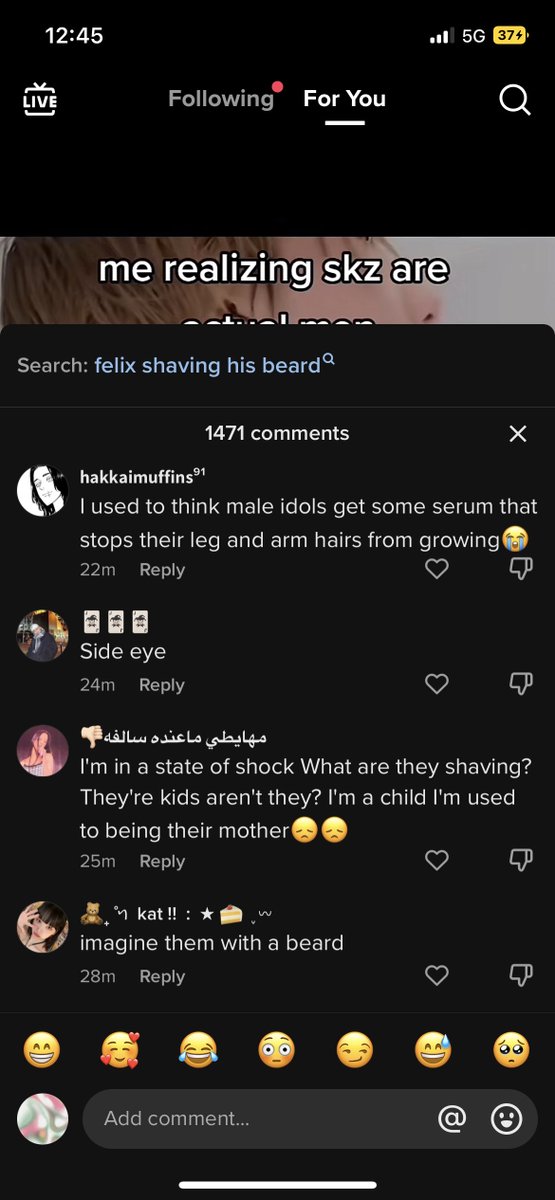Screenshot of a mobile phone screen displaying a social media app interface. 

At the very top, the standard phone icons are arranged from left to right, including the current time, 12:45. In the upper left corner, there is an icon indicating a live session, positioned adjacent to the time. On the upper right corner, the cell phone reception shows three bars with 5G connectivity, and the battery icon indicates 37% remaining charge.

Beneath these standard icons, the app displays two tabs labeled "Following" and "For You," with the "For You" tab being currently selected and underscored. Directly below this, a narrow image spans the width of the screenshot. The image contains the text "Me realizing SKZ R," but the content is cut off at the bottom.

Under the image, there are visible user comments. The first comment reads, "I used to think male idols get some serum that stops their leg and arm hairs from growing." This is followed by a short comment, "Side eye." Another comment states, "I'm in a state of shock. What are they shaving?" The final visible comment is, "Imagine them with a beard."